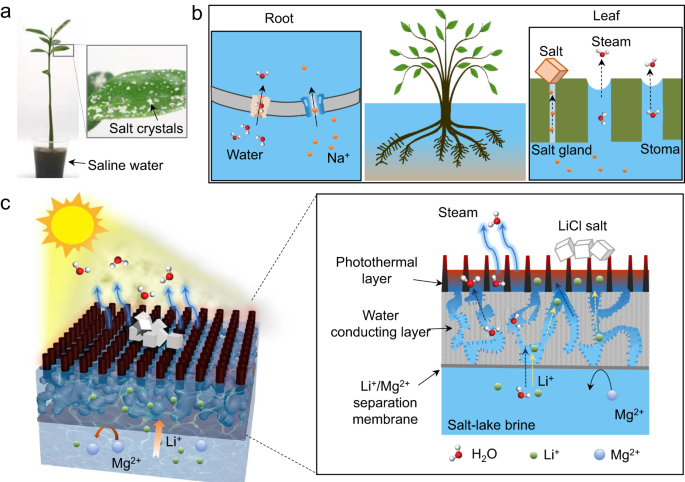This detailed infographic illustrates a scientific cycle involving saline water and a plant's growth. 

In the top left corner, labeled A, there is a detailed image of a potted plant irrigated with saline water. Above the pot, a labeled close-up of salt crystals is depicted, highlighting the saline nature of the water.

To the right, labeled B, the middle section features two diagrams: on the left, a root system showing water and salt absorption, and on the right, the plant’s leaves. This section details the internal process involving roots and leaves where salt, steam, and stoma interactions are illustrated through schematic drawings.

In the bottom half, labeled C, an image of the sun is accompanied by other detailed drawings. These include elements like steam, a photothermal layer, a water-conducting layer, and a separation membrane. Chemical details such as M, G2, LI, LICL, and salt lake brine are also included to elaborate on the processes occurring under sunlight. The illustration is enriched with vibrant blues, greens, yellows, and reds, making it visually engaging despite its complexity.